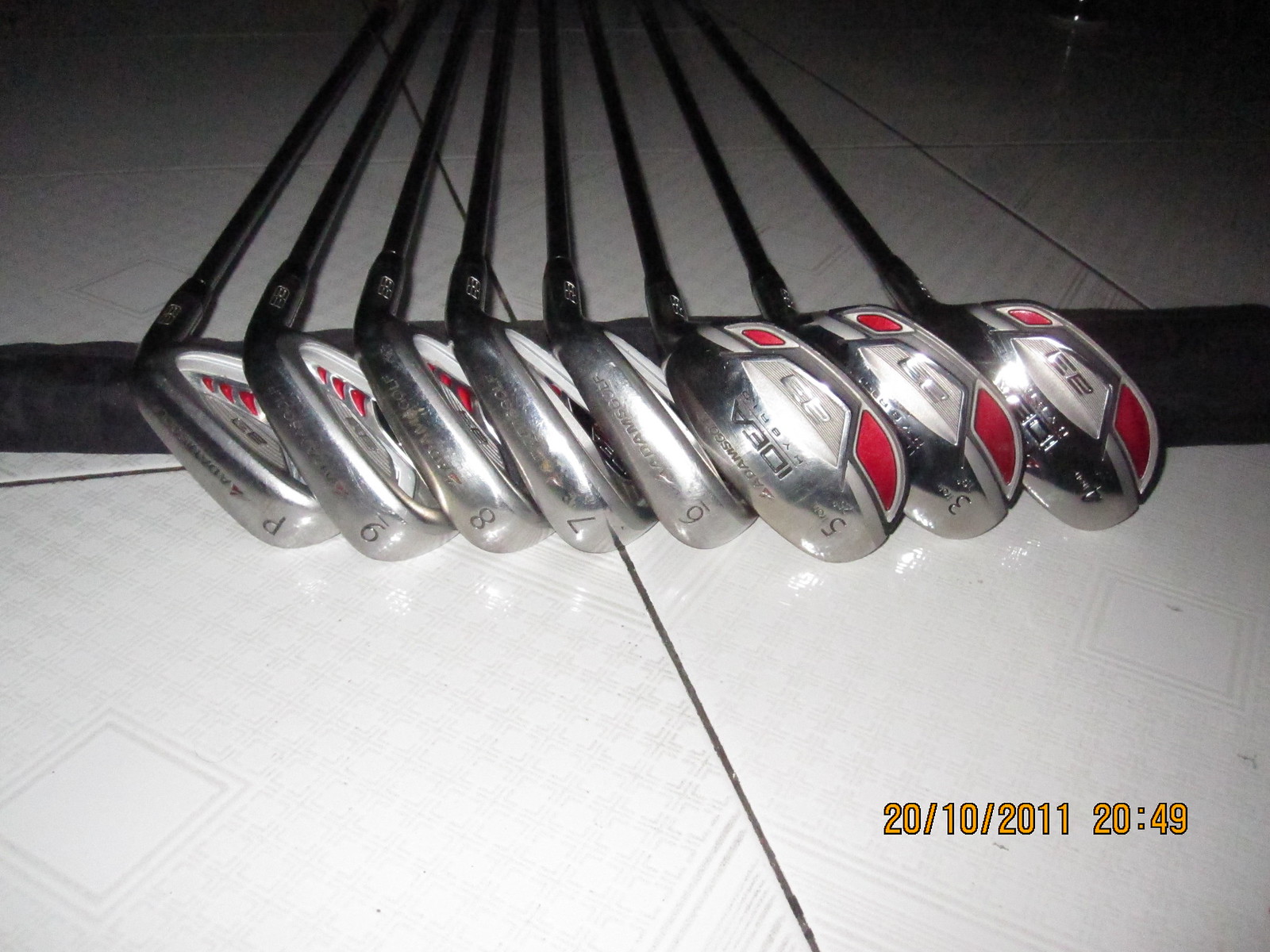The image depicts a neatly arranged set of golf clubs resting on a black and white tiled floor, supported by a rolled-up golf towel. The clubs, belonging to the brand Idea and featuring accents of red against a mostly stainless steel design, appear clean and well-maintained. The set includes various irons numbered P, 9, 8, 7, 6, 5, 4, and 3, along with three drivers numbered 1, 3, and 5, all positioned with their club heads facing towards the camera in an orderly fashion. The clubs' alignment progresses from the smallest club head on the left to the largest on the right, indicating a complete and carefully laid out set. The timestamp on the bottom right of the image reads 20/10/2011 20:49, indicating the photo was taken on October 20th, 2011 at 8:49 PM.